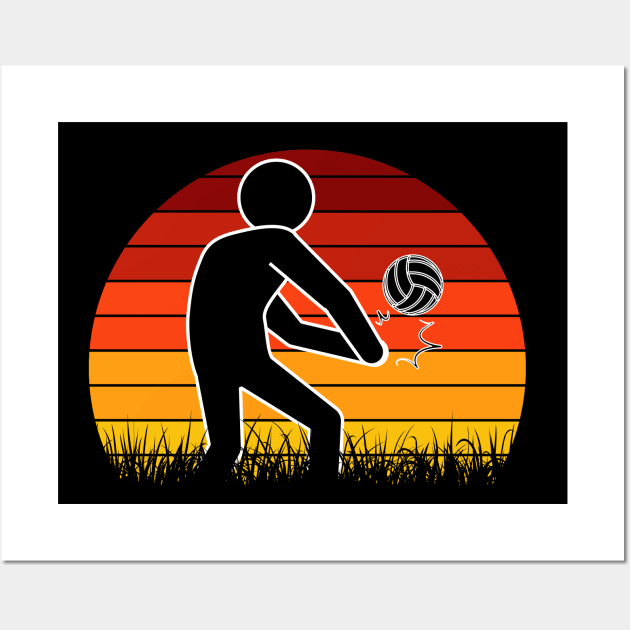This image is a highly stylized vector graphic featuring the silhouette of a person, possibly a man or a woman, hitting a volleyball. The silhouette is entirely black with a distinct white outline, set against a vibrant backdrop. The background forms a gradient that resembles a rising or setting sun, starting with bright sun yellow at the bottom and transitioning through shades of gold, light orange, dark orange, and finally dark red at the top. The action of hitting the volleyball is emphasized by lines indicating movement between the hands of the figure and the ball. The ground beneath the silhouette is depicted as black grass. Surrounding the silhouette is a half-circle, and the entire scene is encapsulated within a box-like frame, adding an additional white box outside that frame in the background. The image conveys a sense of dynamic action and could be used as a sports logo or on athletic apparel.